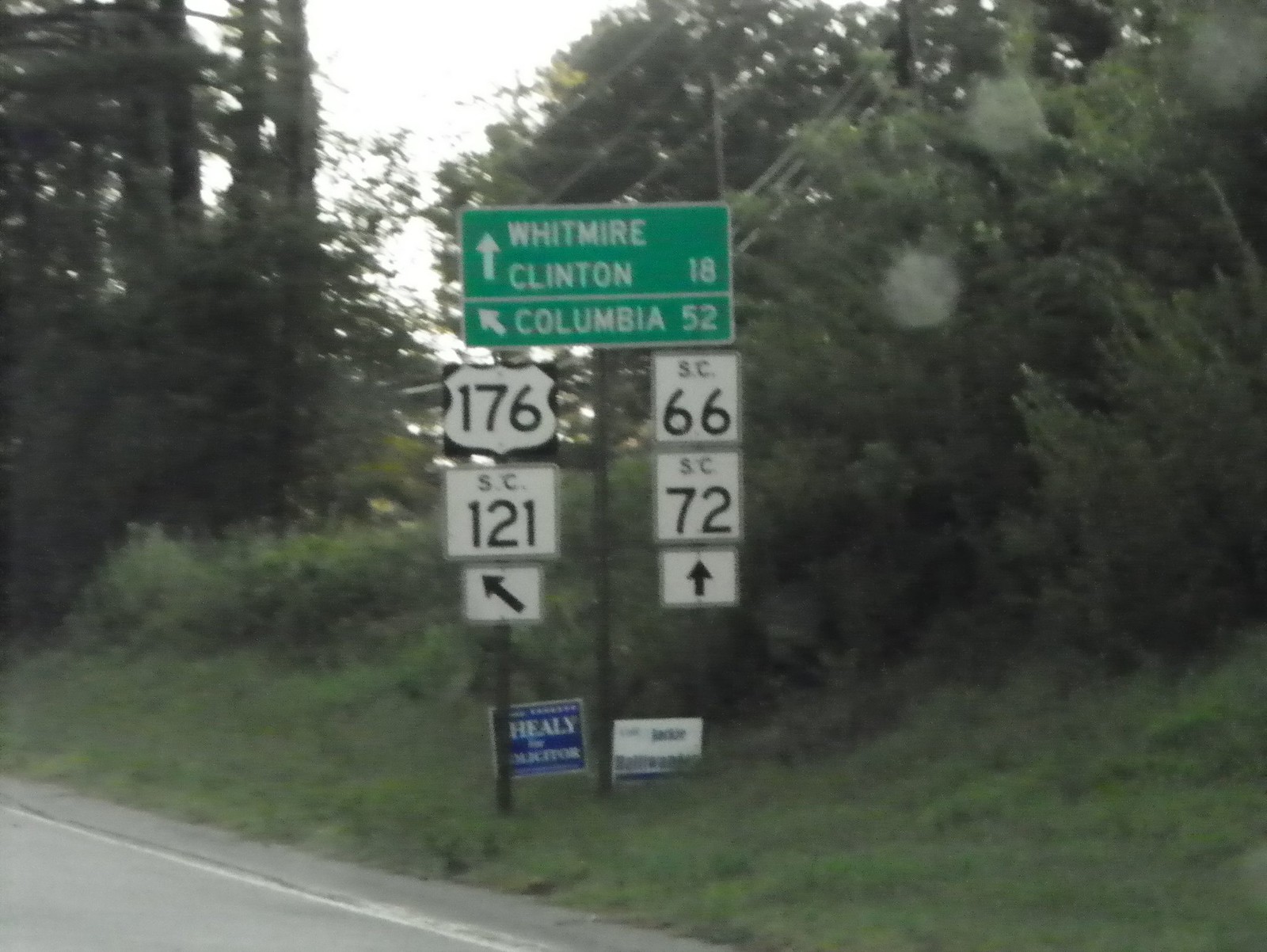In this detailed image, a cluster of navigational street signs stands by the side of a road, which is only partially visible in the bottom left corner, cutting diagonally. Behind the signs, a lush backdrop of trees, shrubs, and grass adds a natural touch to the scene. The signs provide directional information indicating that Whitmire and Clinton lie 18 miles ahead, while Columbia is 52 miles to the left. The presence of signs featuring the "SC" acronym at the top suggests that this location is in South Carolina. 

Prominently beneath the green directional sign, which lists distances to Whitmire, Clinton, and Columbia, there are two SHIELD signs for Route 176 and SC 121, both indicating a left turn toward Columbia. For those continuing straight, SC 66 and SC 72 are the indicated routes. Below this array of official route signs, two additional, less formal signs are visible. One appears to be an election campaign sign supporting someone named Healy, while the other is a homemade, hand-lettered sign whose details are not clearly visible but adds a local, human touch to the roadside tableau.